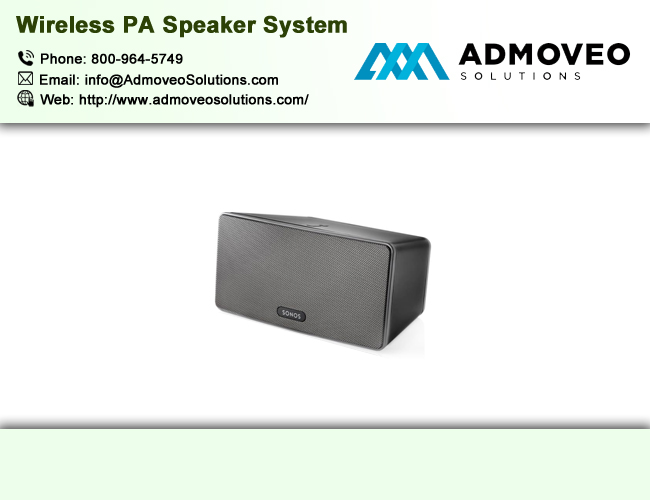This advertisement features a sleek, black rectangular speaker prominently in the middle, labeled with "Sonos." Above the speaker, a banner across the top in green reads "Wireless PA Speaker System." To the right of this banner, a company logo, resembling three unfinished letter A's in blue, represents "AdMoveo Solutions," written in bold black capital letters. Below the text are icons for contact information: a phone symbol with the number 1-800-964-5749, an envelope symbol with the email address info@admoveosolutions.com, and a globe symbol with the website URL http://www.admoveosolutions.com/. The advertisement is framed by a very thin gray border at the top and bottom.